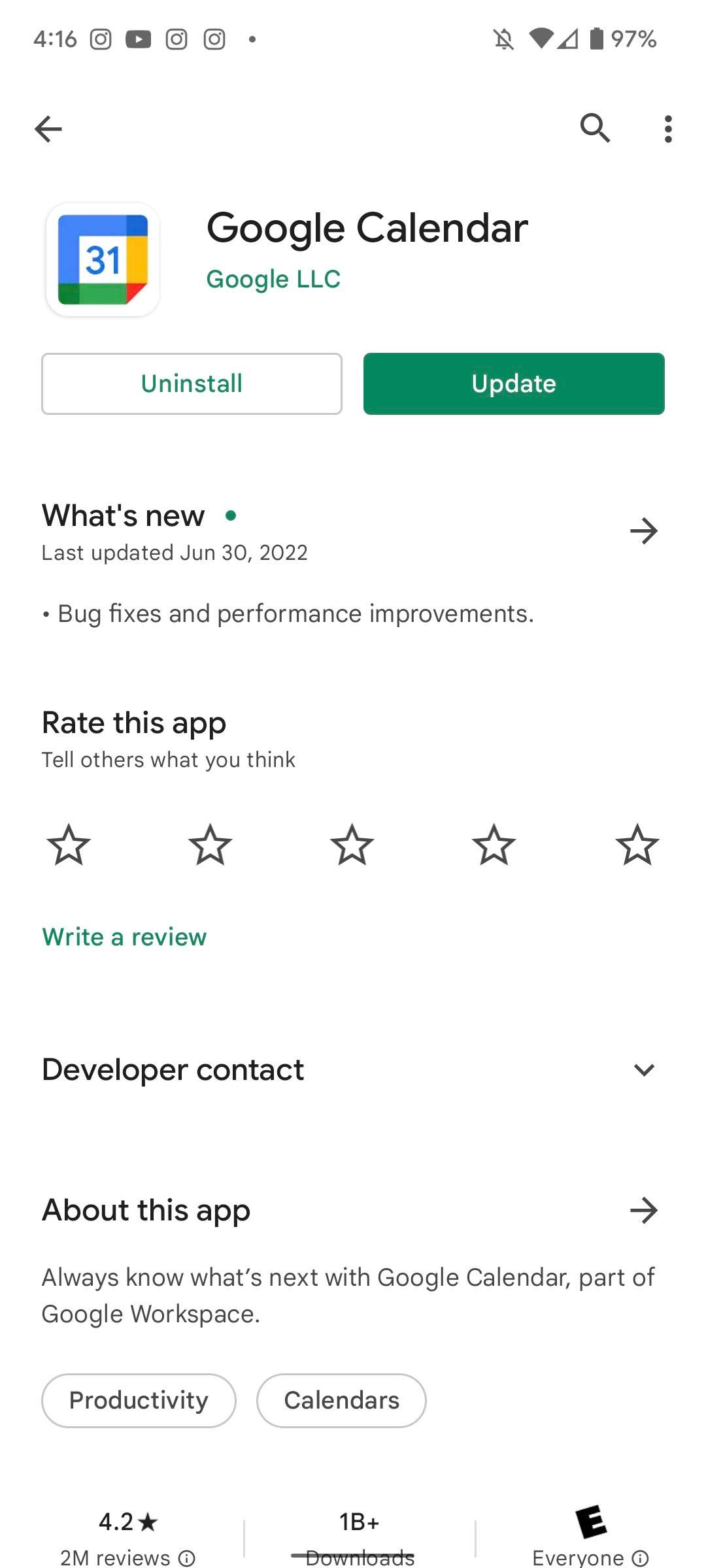In this image, we see the screen of a mobile phone displaying the Google Calendar app page on the Google Play Store. The top left corner of the screen shows the time as 4:16, along with three Instagram notifications and one YouTube notification. On the top right-hand side, icons for Wi-Fi connection, signal strength, and battery level (97%) are visible.

Below these icons, there is a navigation arrow pointing to the left, a search bar on the left side of the screen, and a three-dot menu icon on the right. The main section features the Google Calendar app, with its name displayed in bold black text. To the left of the app name is the app's icon, which consists of a square with green, blue, and yellow borders. The center is white with the number "31" in blue, and the bottom right corner of the square is colored red.

Further down, there are two buttons: "Uninstall" with a white background and "Update" with a green background. Below these options, a "What's New" section highlights that the app was last updated on June 30, 2022, including "bug fixes and performance improvements."

Next, the "Rate this app" section invites users to rate the app out of five stars and write a review, with "Write a review" highlighted in green. Following this is the "Developer contact" section and the "About this app" section, which provide more details about the app. The description reads, "Always know what's next with Google Calendar, part of Google Workspace."

Towards the bottom of the screen, the app's categorical tags are shown: "Productivity" on the left and "Calendars" on the right. Finally, the app's rating summary is displayed: 4.2 stars from 2 million reviews, over 1 billion downloads, and rated "E for Everyone." The entire page is set against a white background.